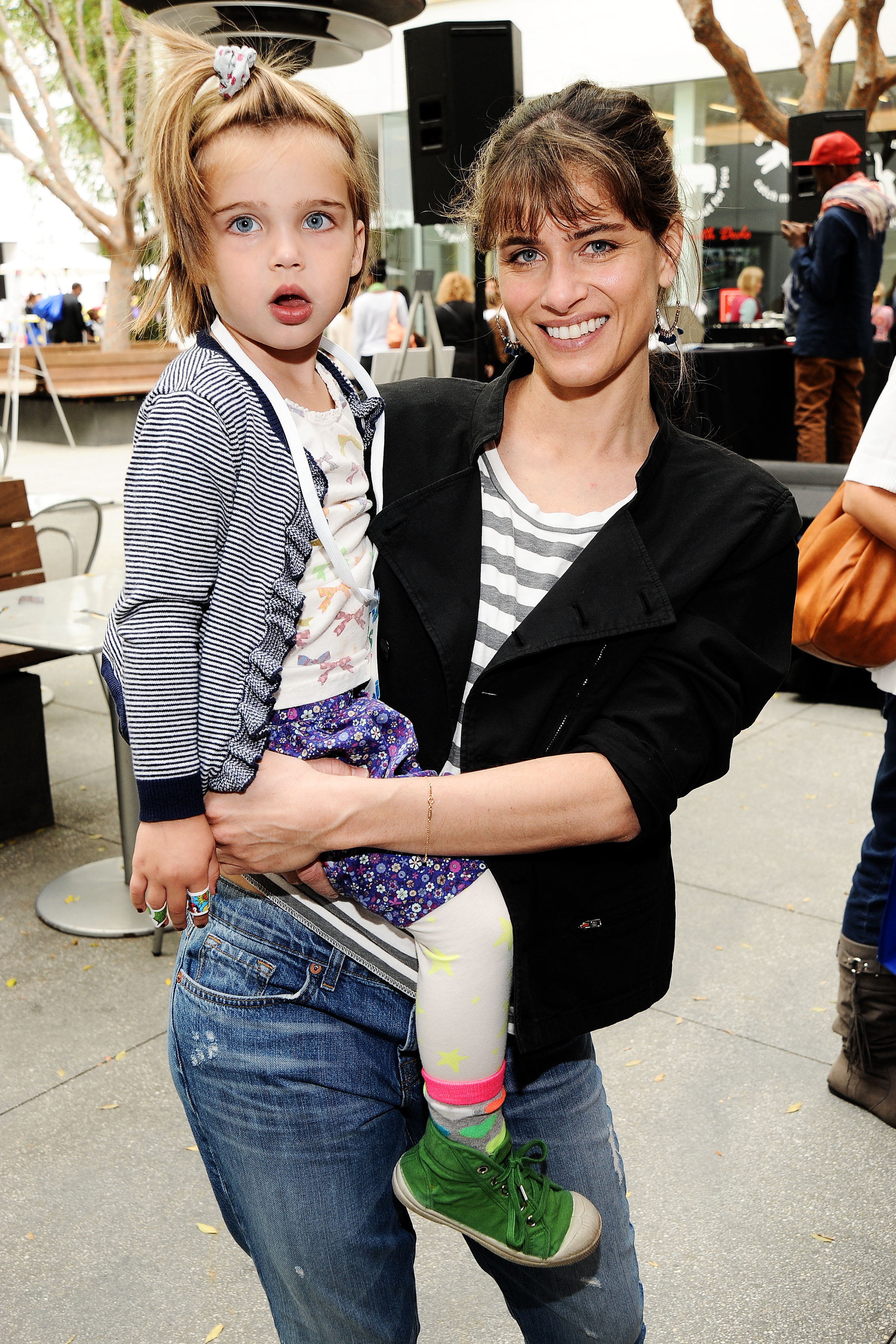In the photo, a white woman in her early 30s with dark brunette hair, styled in a bun with bangs, is holding a young blonde girl with bright blue eyes. The woman is dressed in a gray and white striped shirt, layered under a black cardigan or blazer, paired with medium-wash denim jeans. She wears a warm smile as she looks at the camera.

The little girl, likely her daughter, wears a white shirt adorned with colorful bows—red, blue, green, and yellow—and a black and white striped cardigan. Her outfit also includes a purple skirt or shorts decorated with floral patterns, white leggings with yellow stars, gray socks featuring multicolored hearts, and green sneakers with matching green shoelaces. Her blonde hair is styled in a ponytail on top of her head with a white ruffle. The girl doesn't smile, with her mouth slightly open, giving her a somewhat dazed expression. Additionally, she has two band-aids on one of her hands.

They appear to be standing in a bustling shopping mall, with benches and other people visible in the background. The scene conveys a mix of casual comfort and the vibrancy of a busy public space.